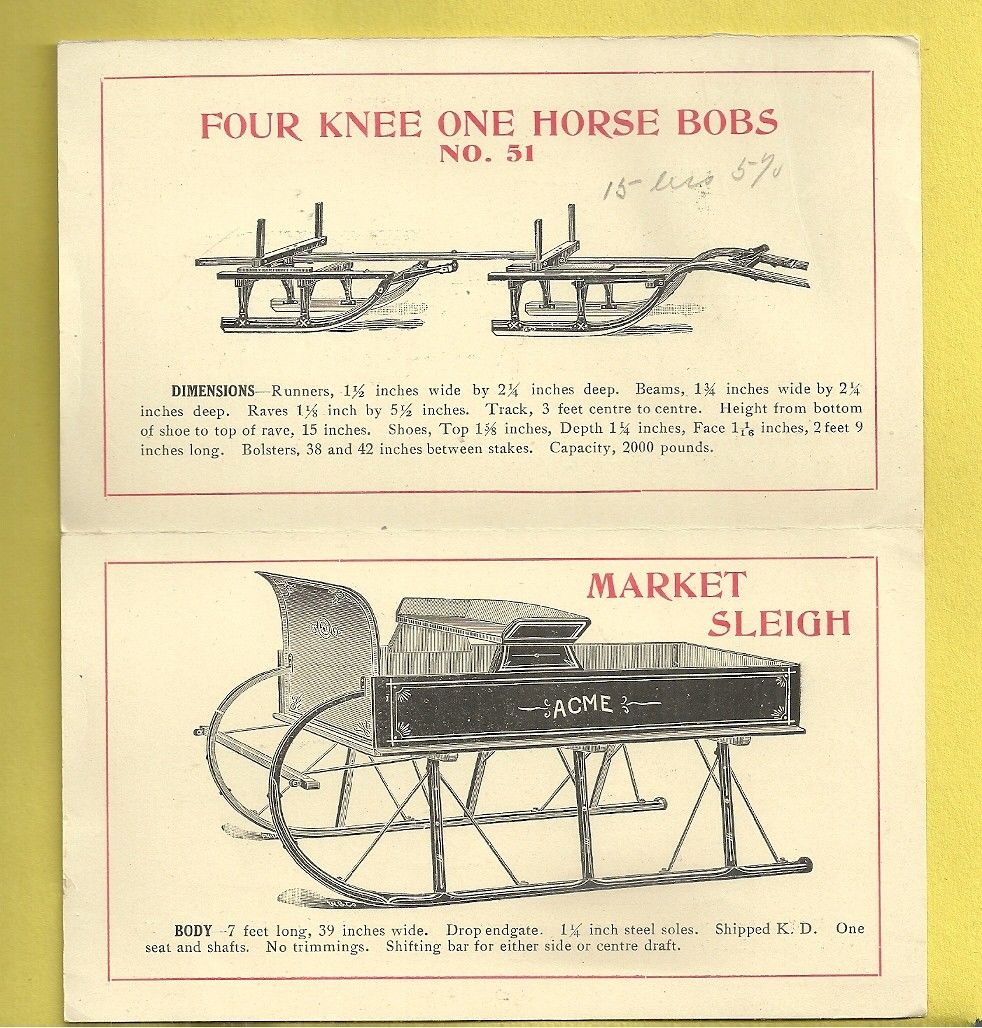This print piece, set on off-white stock, features an advertisement in red and black text with accompanying black drawings. At the very top, bold red text reads "Four Knee One Horse Bobs, No. 51," with indecipherable handwritten notes nearby. Beneath this heading, there is a detailed illustration of two connected snow sleds, reminiscent of bobsleds. The next section, marked again in red with "Market Sleigh by Acme," showcases a larger, black-painted sleigh designed for both a driver and passengers. Notably, the body of this sleigh is seven feet long and 39 inches wide, sporting "Acme" on its side. Dimensions of the runners, specified alongside, measure one and one-half inches wide by two and a quarter inches deep, adding to the technical details provided.